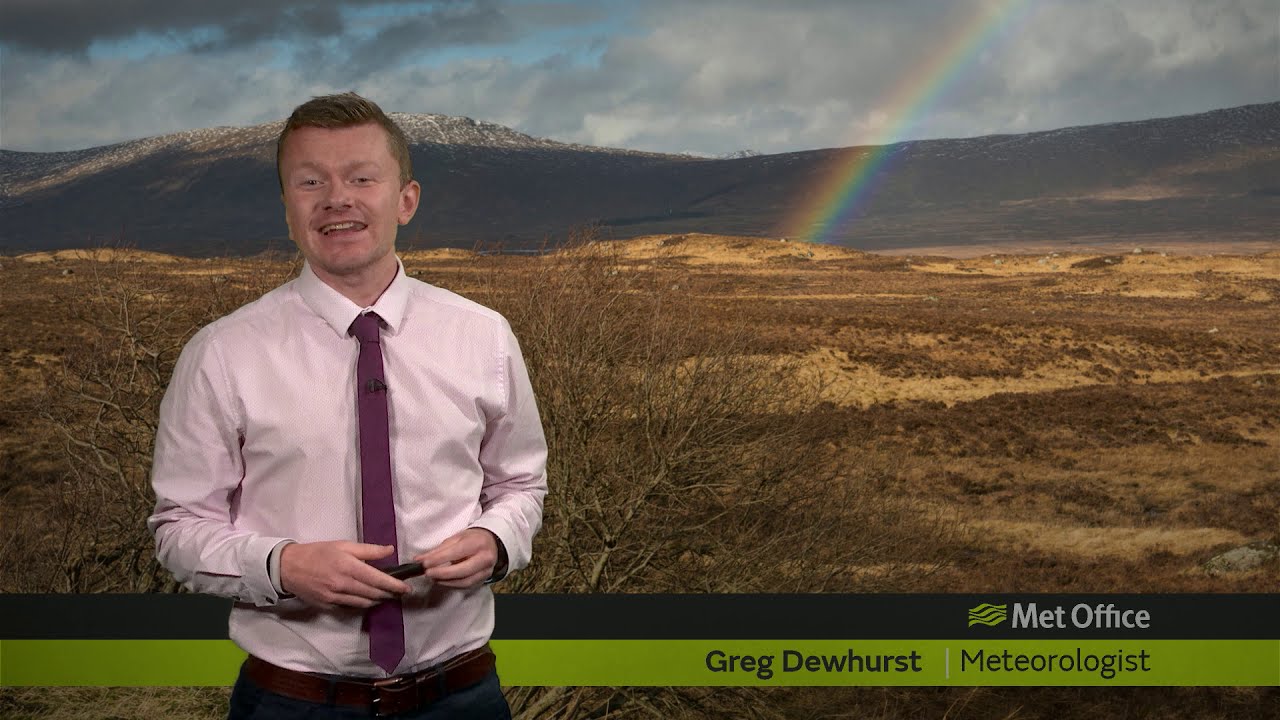In this image, a meteorologist identified as Greg Dewhurst stands in front of a green screen displaying a barren landscape. Greg Dewhurst, as indicated by the overlay text "Greg Dewhurst Meteorologist" in black font at the bottom of the screen, is on the left side of the picture. The bottom of the screen also features green and black stripes, accompanied by a "Met Office" label in white font with a green-striped icon to its left.

Greg, a young white man likely in his early 30s, sports short brown hair neatly slicked to the right with a clean cut on the left side. He wears a white or pinkish long-sleeve button-down shirt paired with a burgundy or purple tie, which has a small black microphone clipped to it. He also has on a brown belt and blue or gray pants. His hands are positioned in front of his midsection, clasping a black clicker or similar device. He is smiling slightly.

The background scene presents a desolate, dry dirt area dotted with leafless shrubs and trees, stretching out towards a shadowy mountain range with patches of snow on the peaks. A mostly cloudy sky looms above, filled with gray and black rain clouds interspersed with subtle hints of blue and white clouds. On the right side of the image, a vivid rainbow emerges from the barren land, arching halfway upward into the sky in a spectrum that includes shades of red, yellow, green, blue, and sometimes purple. Overall, it captures the essence of a weather report being broadcasted from a makeshift desert setting.